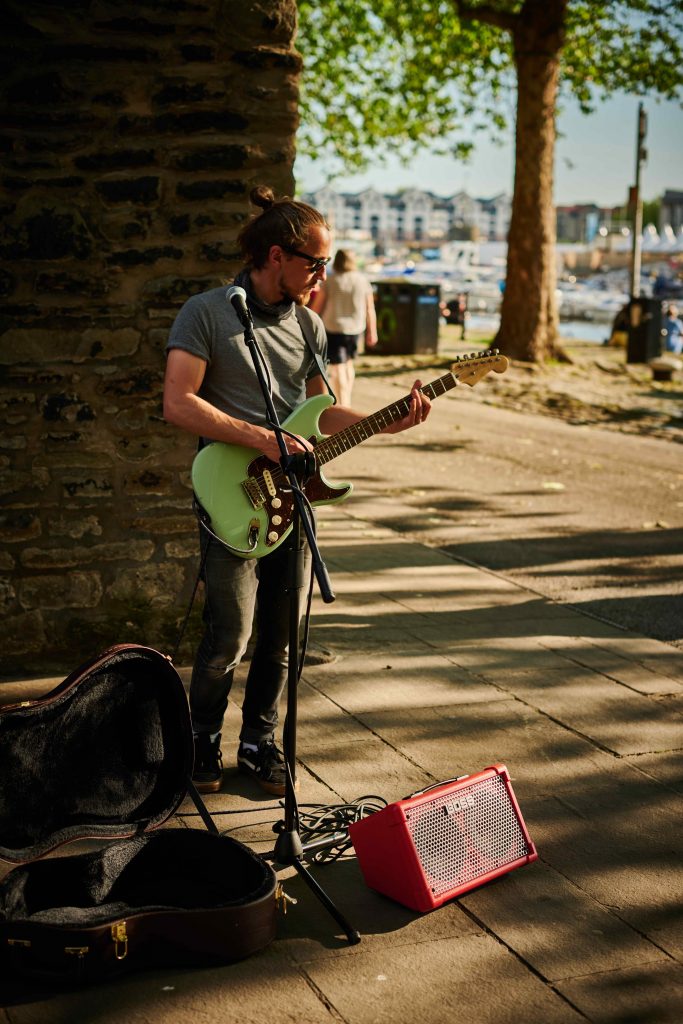This vivid daytime street scene captures a live outdoor performance by a light-skinned man playing a green electric guitar. He stands beside a dark brown brick wall, his hair tied up in a bun, wearing a short-sleeved gray t-shirt and matching gray pants. A pair of sunglasses shades his eyes as he plays, positioned in front of a black microphone stand. At his feet lies an open brown guitar case with a black velvet interior, presumably for collecting donations, indicative of his busking activity. Beside the case, there is a small red Boss sound system. The cement sidewalk, detailed with stone tiles, stretches along the foreground of the image. In the background, slightly out of focus, are apartment-like buildings, a tree, and other passersby. The scene exudes the vivacity of a beach community, blending elements of urban and coastal atmospheres.